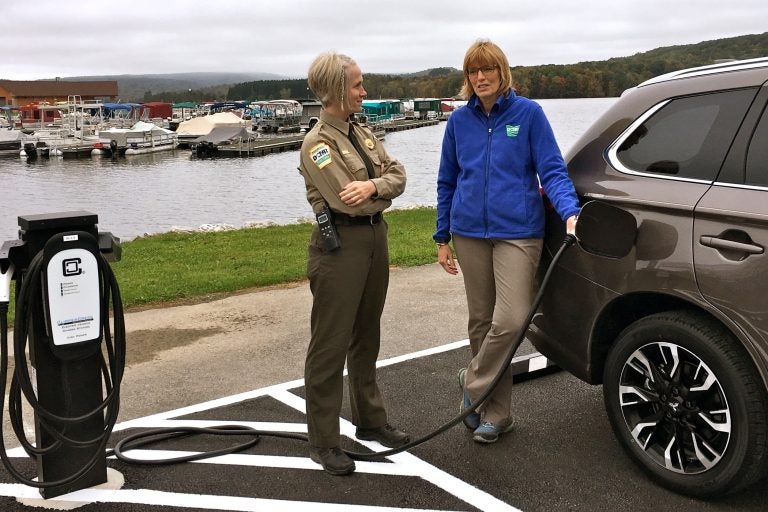In the photograph, two women stand in front of an electric charging station at a scenic port filled with boats. One of the women, who appears to be in her 40s, has short blonde hair and is wearing glasses, a blue jacket, and tan pants. She is in the process of charging her bronze-colored electric SUV. Beside her is a policewoman with short blonde hair, dressed in a light tan police uniform with a badge and a walkie-talkie attached to her belt. The policewoman is also wearing dark brown pants and shoes. The background features a clear white sky, green hills, and buildings, creating a picturesque setting around the lake or river with docks lined with boats. The irregular concrete street where the women stand is marked with white lines, adding to the detailed outdoor scene.